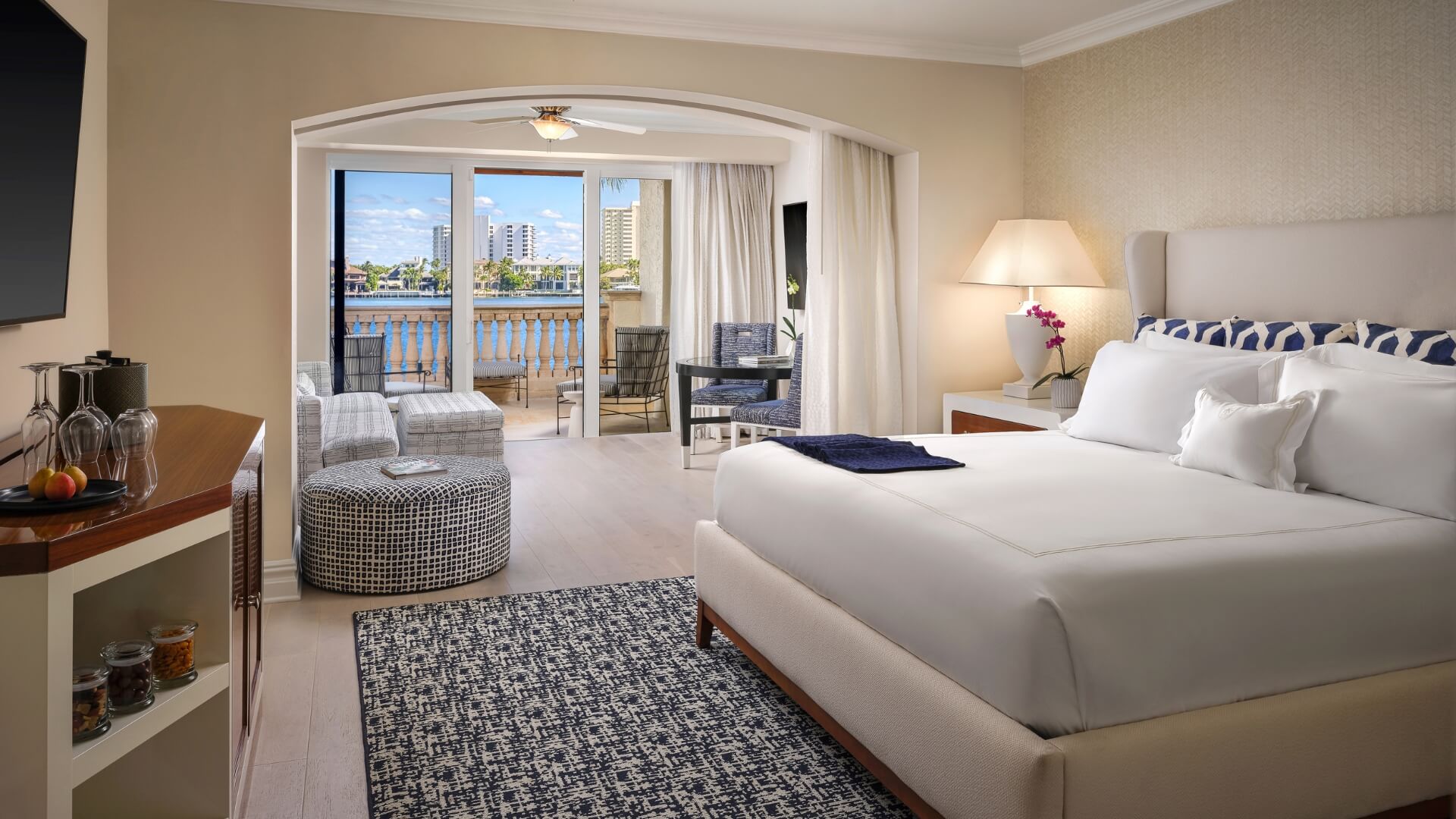The image depicts a luxurious master bedroom, likely in a high-end hotel suite, featuring ivory walls with white trim and a white ceiling. The centerpiece is a king-sized bed with a tightly tucked, white comforter. The bed is adorned with six white pillows and additional blue and white cushions, complemented by a beige upholstered headboard. A gray and white area rug extends from under the bed. To the right is a lamp and a vase with red flowers.

Opposite the bed, a large flat-screen TV is mounted on the wall, above a cabinet holding wine glasses, an ice bucket, and several jars of peanuts on a side cabinet. Beneath the cabinet, three candles are arranged on a shelf. A circular stool provides additional seating nearby.

The room features an arched doorway leading into a cozy sitting area, furnished with a gray chair, a desk, a large black-and-white ottoman, and a cream and gray oversized chair with a footrest. This space transitions to a balcony through sliding glass doors. 

The balcony itself is fitted with multiple seating options, including chairs with blue backs and another with a hollow design. The balcony overlooks a serene body of water—be it a river, lake, or something similar—and offers a picturesque view of distant skyscrapers.